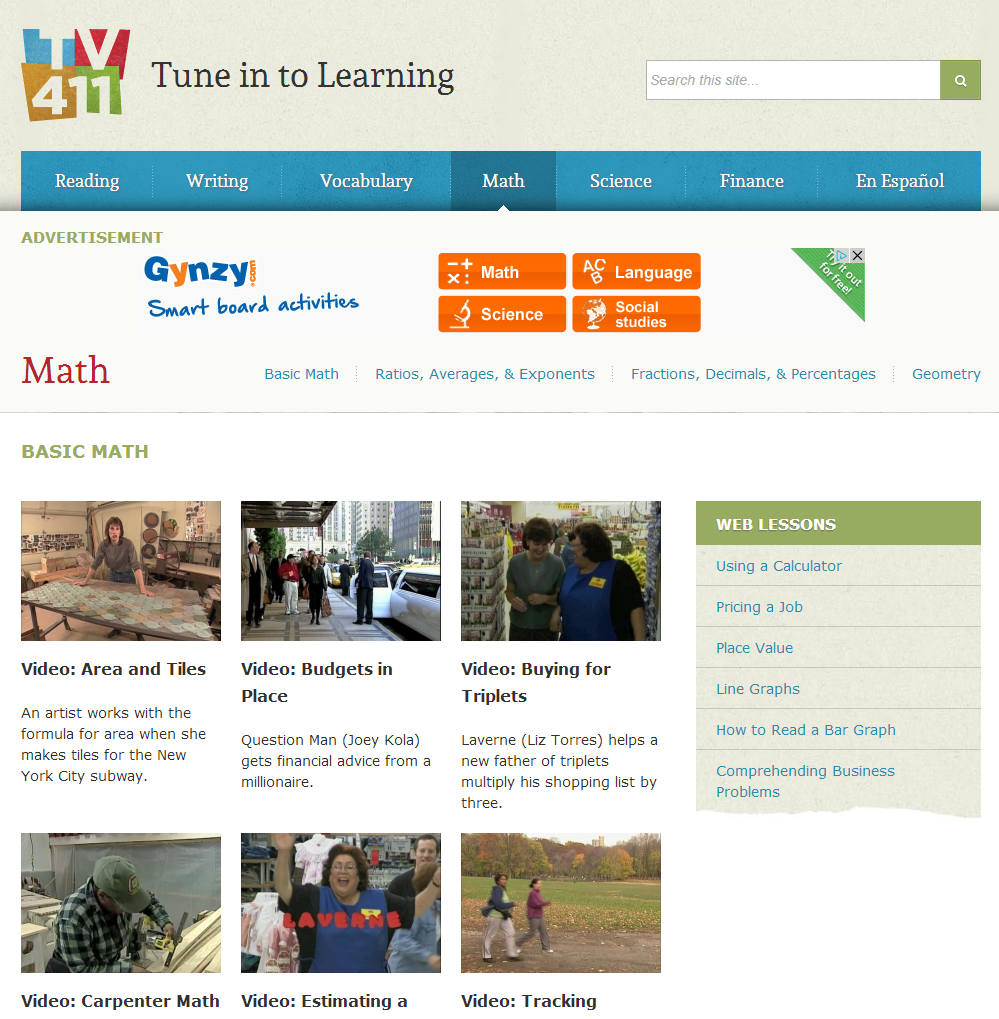The top section of the image features a gray background. In the upper left corner is a square comprised of four colored segments: blue, red, orange, and green, with the text "TV411" in white inside the square. Adjacent to this, in black text, are the words "Tune into Learning."

On the right side, there is a gray search bar labeled "Search the Site" along with a green square containing a white magnifying glass icon.

Below this, a blue section with slightly darker blue text lists the categories Reading, Writing, Vocabulary, and Math. Subsequent categories in the same text color include Science, Finance, and Español.

An advertisement for "Smart Board Activities" is also present, though it is of less interest. Beneath this ad, there is black text divided into several parts with white spaces interspersed:

- The first section, labeled "Math," lists Basic Math, Ratios, Averages, Exponents, Fractions, Decimals, Percentages, and Geometry.
- Green text on the left reaffirms Basic Math.

Following these sections are generic stock photos. Underneath, black text titles the video listings and gray text provides descriptions:

1. Title: "Video: Areas and Tiles"
   Description: "An artist works with a formula for the area while she creates tiles for the New York subway."

2. Title: "Video: Budgets and Place"
   Description: "Question Man Joey Cola receives financial advice from a millionaire."

3. Title: "Video: Buying for Triplets"
   Description: "Vaza Liz Torres assists a new father of triplets in multiplying his shopping list by three."